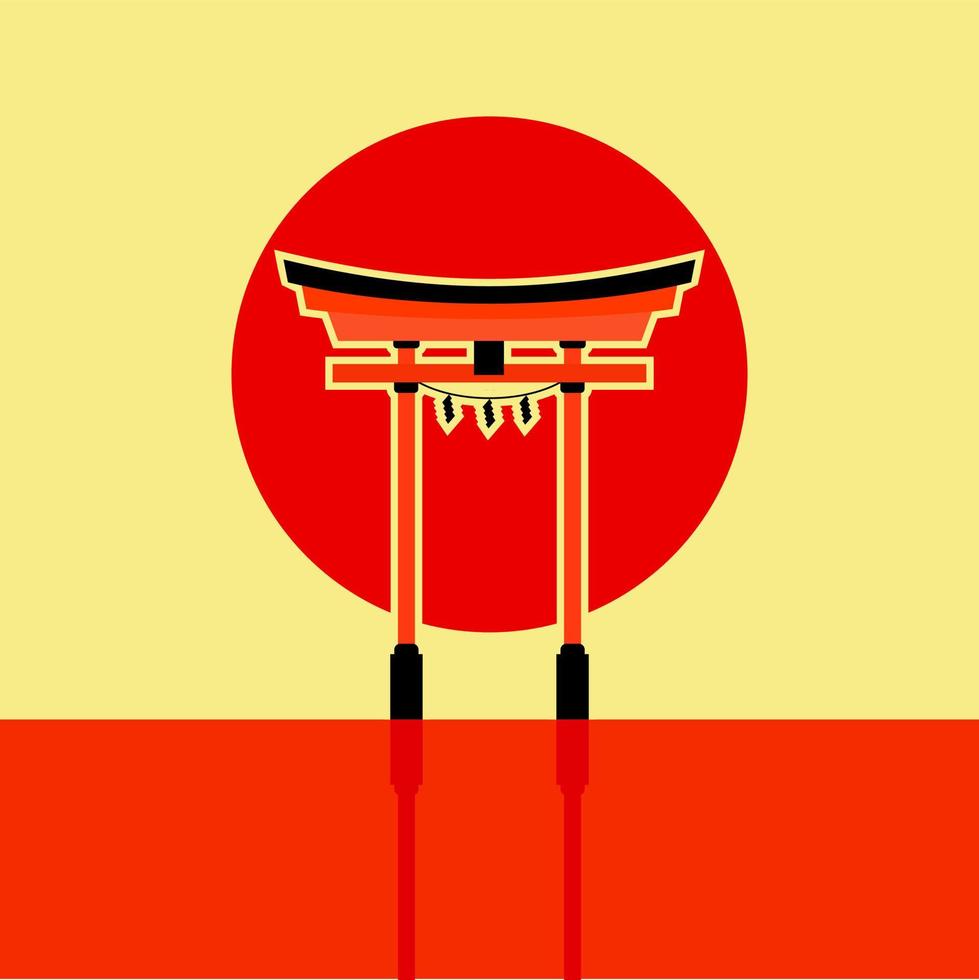The image is a detailed illustration featuring a traditional East Asian structure, possibly inspired by Chinese or Japanese architecture. The backdrop primarily consists of a large, light yellow rectangle, with a dominant red circle centered within it, reminiscent of the sun or moon. At the bottom of the image, across its width, lies a thick, bright red banner. From this red base, two vertical poles rise upwards, framed in black color at their bases, and supporting a horizontal crossbeam with a slightly curved top. This top section, resembling the roof of a pagoda or a pergola, has a black, upward-curving eave. Between the vertical poles, just below the crossbeam, a string is stretched with three hanging objects, likely lanterns, adding to the decorative effect. Overall, the orange and black elements contrast vividly against the yellow and red background, creating a visually striking emblematic image.